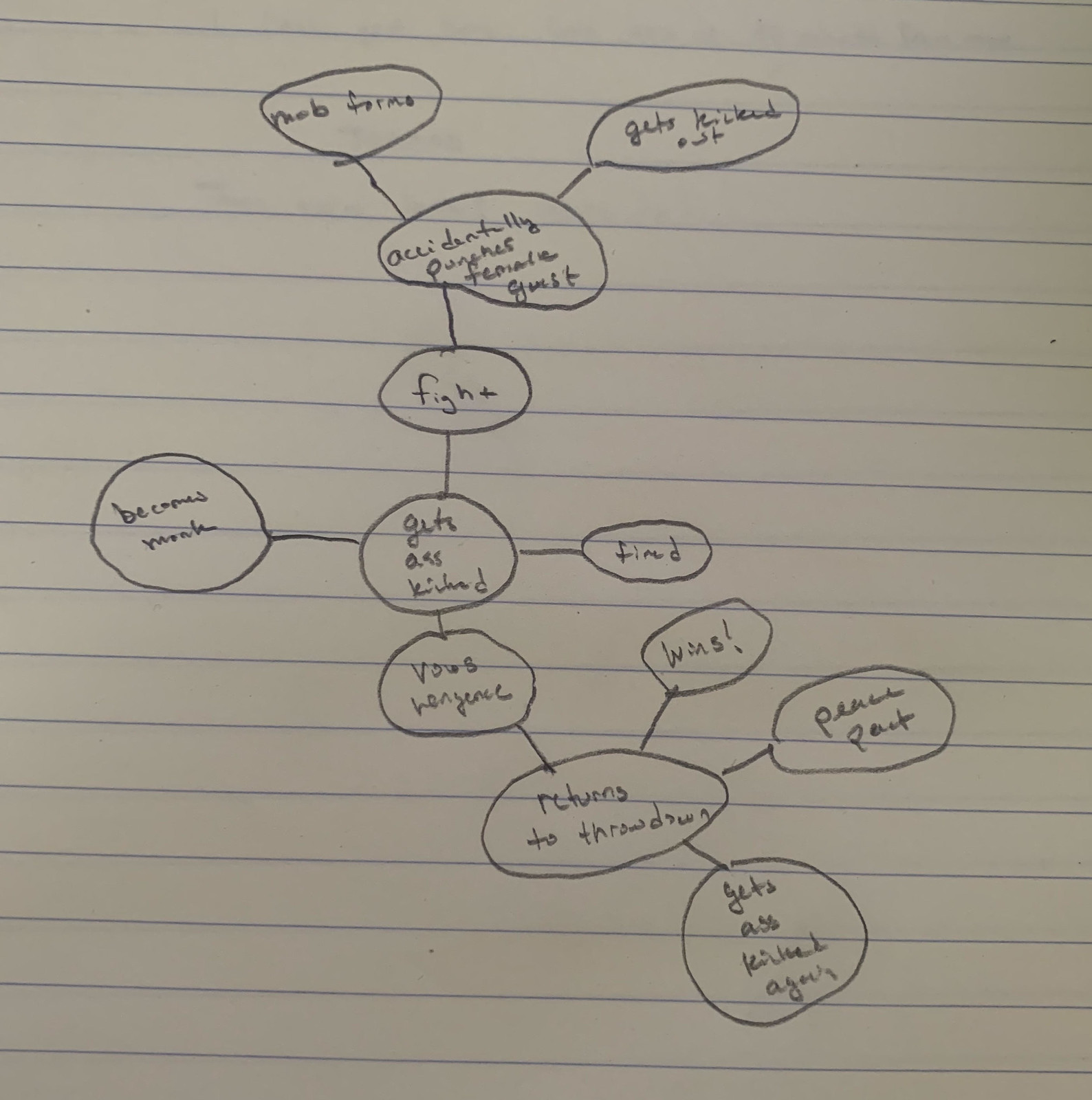The image is a detailed pencil drawing on notebook paper, with the blue horizontal lines of the paper visible throughout. The drawing depicts a series of interconnected circles, arranged in a vertical flowchart that spans from the top to the bottom of the page. 

At the top, part of the image appears to show partially legible text within a circle, seemingly labeled "Mob Forms." Nearby, to the right, is an additional circle that is slightly offset and connected by a line, possibly referring to an error or deviation, as indicated by fragmentary text. This leads to another circle labeled "Accidentally," though the full text within the circle is unclear.

Continuing down, a clear connection leads to a circle labeled "Fight." From there, a line connects to a circle reading "Gets Ass," but the bottom portion of the text is unreadable. This circle branches into two directions: the rightward circle is marked "Find," and the leftward circle seems to read "Becomes," with the subsequent word illegible.

Further down, a linear progression links to a circle labeled "Vows Vengeance," followed by another circle that states "Returns to Throw Down." Above this central circle is one labeled "Wins," and to the right is another circle potentially labeled "Peace, Past."

Finally, at the very bottom of the drawing, there is a circle with the text "Gets Ass Kicked Again."

The overall diagram resembles a complex flowchart of events or actions, though some of the specific details within the circles are difficult to decipher.